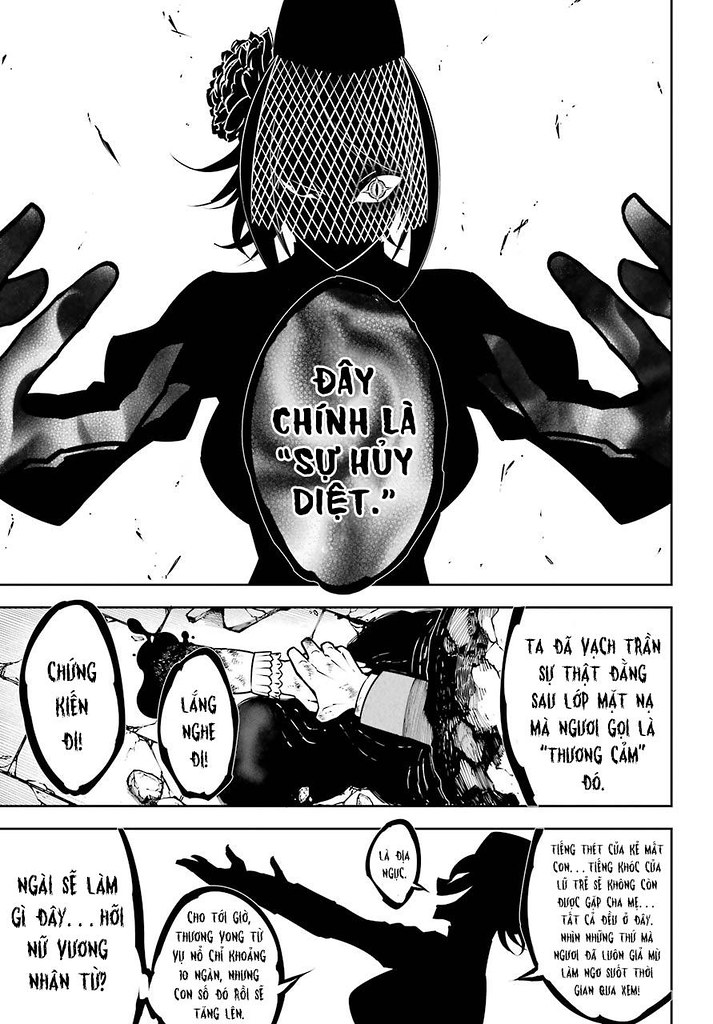This is a three-panel manga comic rendered in black and white. The top panel, which occupies half of the image, prominently features a woman shrouded in shadow and wearing a mesh veil that covers her face. Only one of her eyes is visible, exhibiting a sinister star-shaped pupil, while the other eye is nearly closed. A black rose adorns the left side of her head. She extends her hands forward in a menacing, grasping gesture as if casting a spell. A text bubble next to her reads, "Dei Chin La Se Hai Diet," written in Vietnamese.

The middle panel showcases a desperate scene where multiple arms, seemingly crushed under rubble, reach out. One bloodied hand grasps a severed woman's arm, which lies in a pool of blood.

In the bottom panel, the silhouette of what appears to be the same woman from above is shown from a side profile. She is depicted laughing maniacally, her arms raised high in a malevolent pose. Her expression is heinous, evoking a creature of pure darkness. Speech bubbles with Vietnamese text accompany her menacing outline. The entire comic exudes an eerie, grim atmosphere.